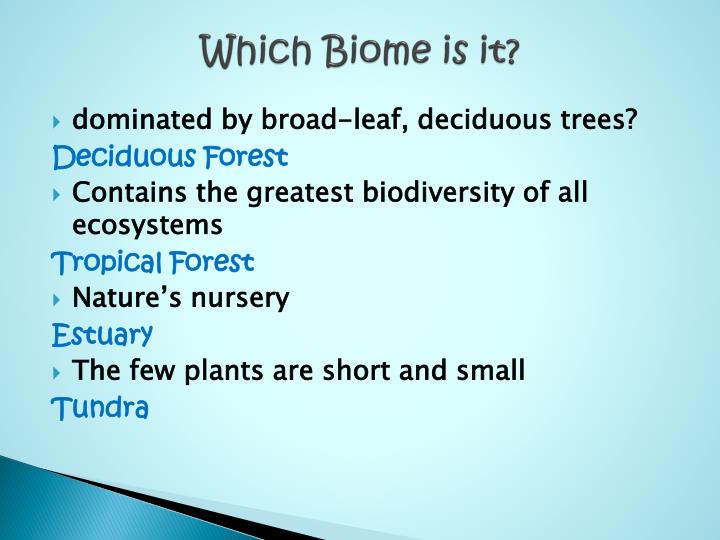The image has a light blue background with a darker blue section in the bottom left corner. The central text is a title and several bulleted points. At the top, in black letters, the title reads "Which Biome Is It?" Below the title, a series of questions and answers are listed. The first question asks, "Dominated by broad-leaf, deciduous trees?" in black letters, and the answer below it is "deciduous forest" in blue. The next bulleted question in black states, "Contains the greatest biodiversity of all ecosystems?" followed by the answer "tropical forest" in blue. The subsequent bulleted question, "Nature's nurseries?" in black is answered by "estuary" in blue. Lastly, the question "The field plants are short and small?" is in black, with the answer "tundra" in blue.